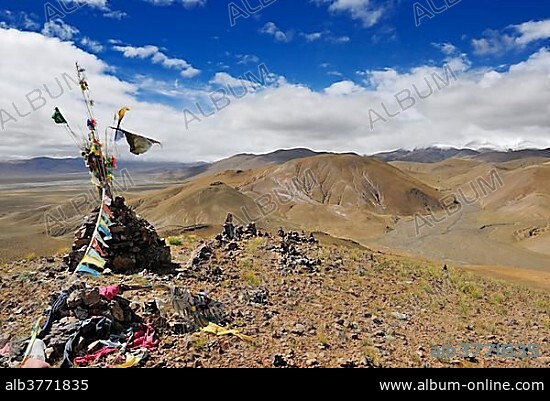In this image, protected by a significant 'album' watermark from www.album-online.com with the name alb3771835, a desolate and rugged landscape stretches into the distance, dominated by small, brown, dirt mountains under a vivid blue sky streaked with clouds. In the foreground, a stone mound stands prominently, adorned with a bouquet of flowers and a handmade flag banner, colorful yet hard to distinguish in detail. The banner stretches from the stones up to an object, potentially a makeshift tent or structure, partially out of frame and attached by a stream of triangular flags. The scene evokes a remote, arid environment, possibly somewhere like Nepal, notable for its striking natural beauty and its appeal to adventurous hikers seeking far-off places.